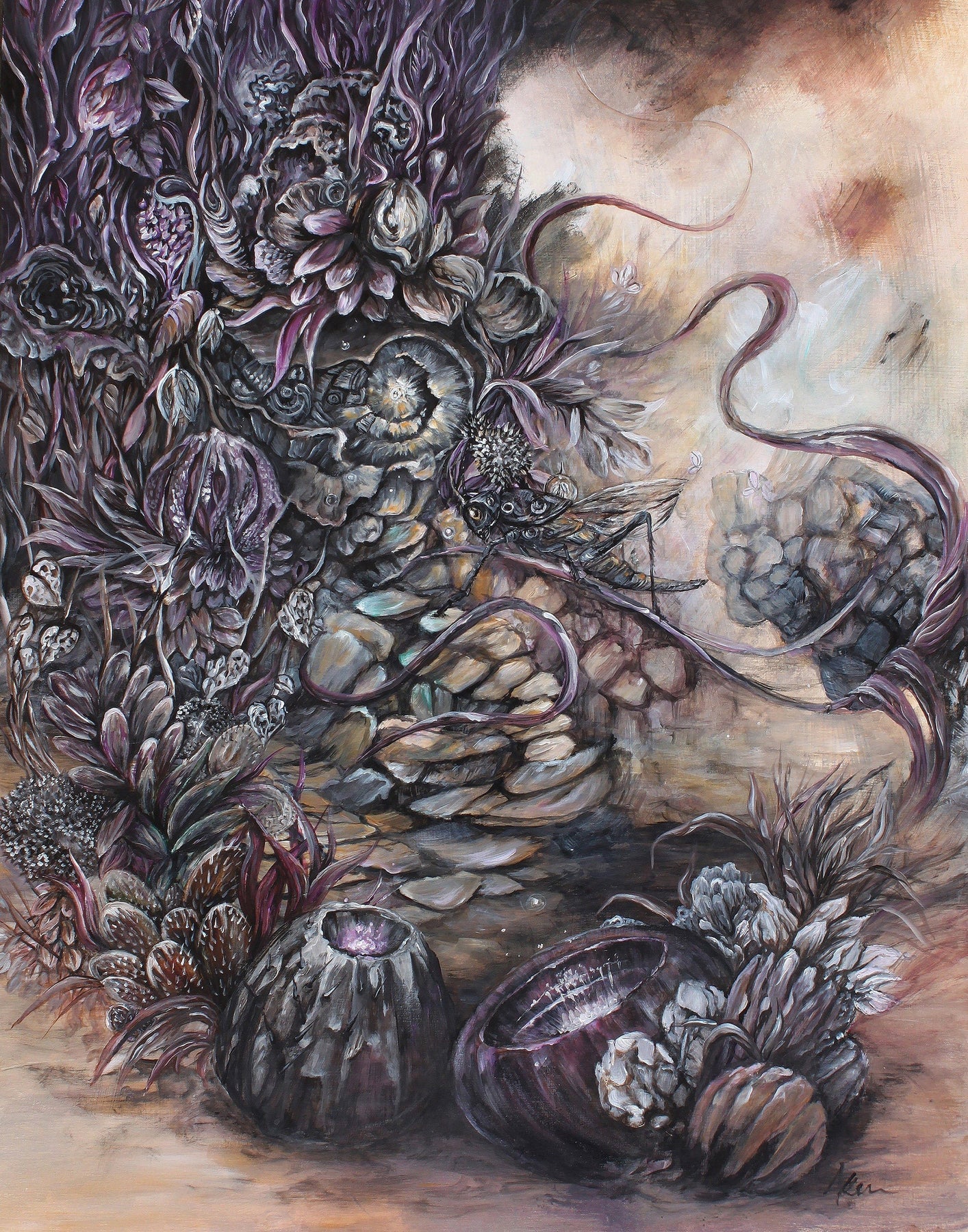This oil painting portrays an otherworldly scene brimming with alien-like plant life. The composition is dominated by vibrant purples and blues, with sporadic bursts of orange enhancing the surreal atmosphere. The artist's visible brush strokes bring texture and depth to the flora that populate the scene. These plants exhibit diverse forms, ranging from petals and tendrils to bulbous shapes. Noteworthy among them are two coconut-like structures near the bottom center; one, slightly to the left, reveals a glowing purple interior, while another, to its right, mirrors this luminescence with a broader opening. Nearby, other shapes reminiscent of chestnuts or pine cones further enrich the scene. The plants predominantly cluster in the top left corner, appearing to grow upwards like a living wall, while others spread across the brown earth below. The background blends shades of tan and light brown, accentuated by visible brushwork that intermingles with the orange hues. The mix of floral elements, muted yet varied colors including deep magenta, dark greens, and light ivory, creates a mesmerizing tapestry that spans about two-thirds of the canvas, giving the painting a vibrant, organic feel despite its extraterrestrial motifs.